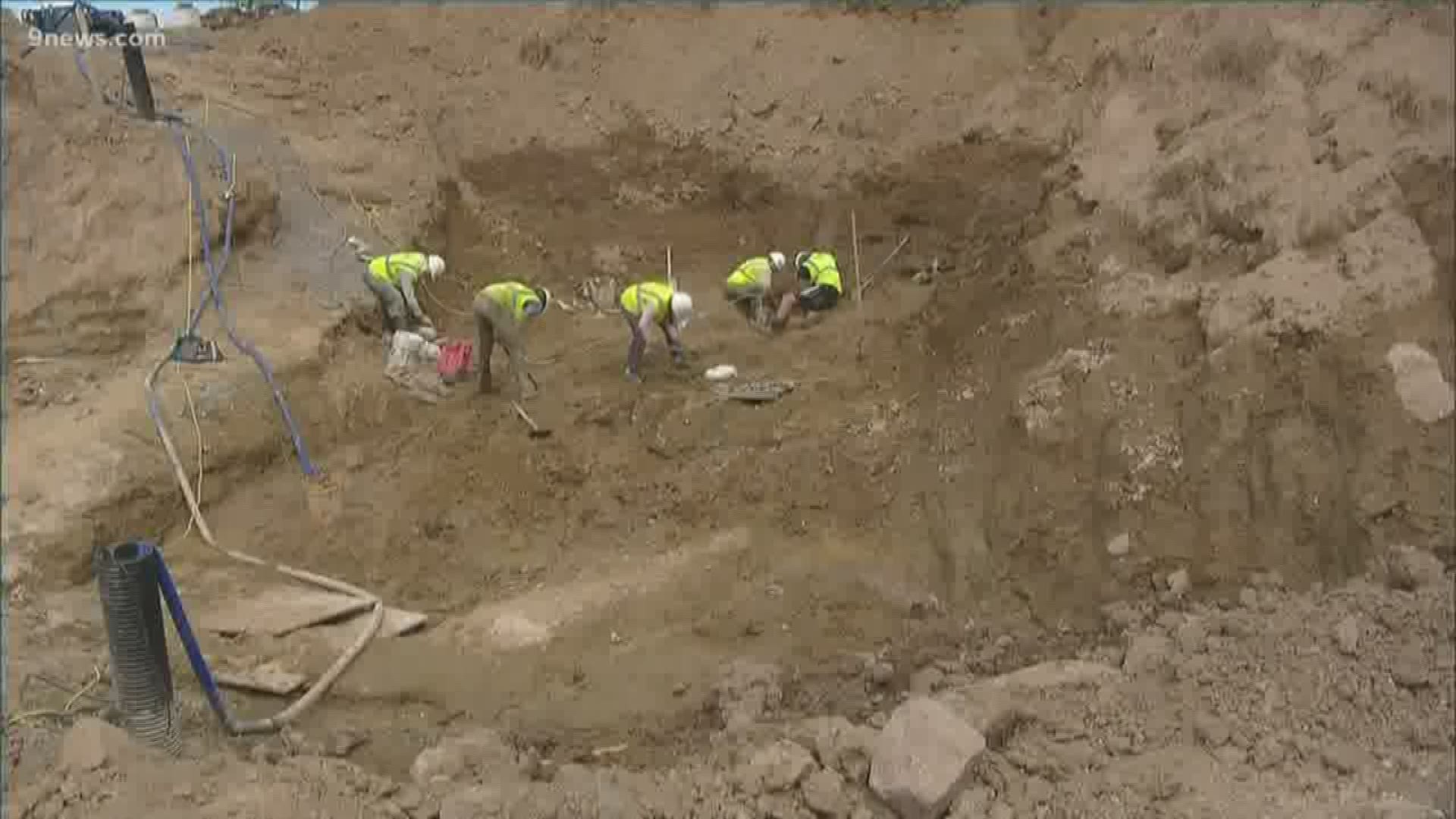The photograph from 9news.com captures a group of five men working on a large, dirt-covered hillside. Each man is equipped with a bright yellow-green safety vest and a white hard hat. Three of the men are standing, bent over as if inspecting or retrieving something from the ground, while the other two are seated further back, similarly engrossed in the soil, possibly digging with their hands. The background features the brown clay color typical of a sand or gravel pit, contrasting with long blue tubes running down the hill, possibly for water or another utility. The workers' focus is evident, though the exact nature of their task remains unclear, with possibilities ranging from rescue efforts after a disaster to routine construction activities. The absence of emergency vehicles suggests it's likely a non-urgent assignment. Shovels and a sledgehammer are scattered around, indicating heavy manual labor.